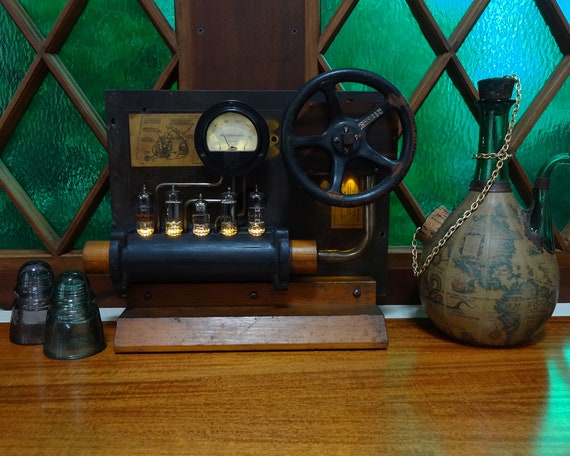This indoor scene captures an eclectic collection of vintage and mechanical objects arranged on a light brown wooden table. Dominating the center is a rectangular contraption that combines elements of both a cash register and an engine. This intriguing piece features a black metal steering wheel mounted on its right side, a speedometer in the center, and a series of pistons connected to a black cylindrical element below. The base is constructed from wood, providing a sturdy foundation. Adjacent to this machine, on the right, sits a vintage-looking glass coffee pot adorned with antique maps on its round base and a tall spout topped with a chain hanging into another spout at the bottom. On the left side of the mechanical device, two inverted glasses, resembling salt and pepper shakers, can be observed. In the backdrop, a wood-framed panel with green glass arranged in a diamond pattern adds a rustic charm to the scene. Scattered throughout are other intriguing items, including green conical glass objects reminiscent of telephone pole insulators on the left and a gourd-shaped green glass object on the right. The arrangement of these unique pieces evokes a sense of historical curiosity and mechanical innovation.